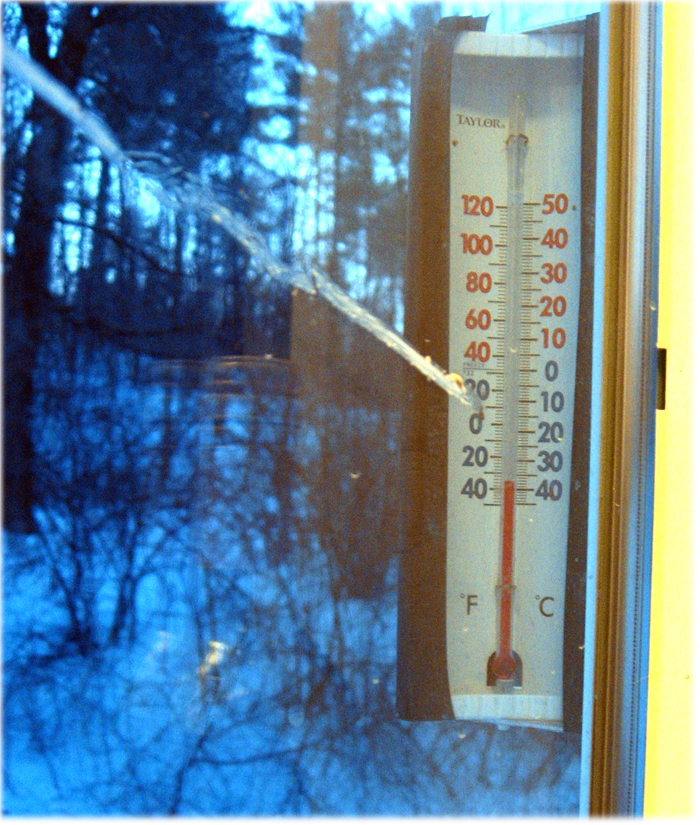This photograph captures a close-up view of a vertical outdoor thermometer attached to a window. The image is taken from inside the house, looking out through the glass. The thermometer, prominently labeled "Taylor," features an outer casing of brown plastic with a white plastic interior. It is designed with two scales: Fahrenheit on the left and Celsius on the right. The Fahrenheit scale, marked with an "F," ranges from 120 degrees down to 40 degrees below zero, while the Celsius scale, marked with a "C," spans from 50 degrees to 40 degrees below zero. The lower part of the thermometer contains a clear glass bulb filled with red liquid, which currently indicates a temperature around 35 degrees Fahrenheit.

Beyond the thermometer, the background reveals a picturesque winter scene. The ground is covered in snow, the sky is a crisp blue, and the leafless trees stand bare against the cold. However, this backdrop is somewhat blurred, keeping the focus on the thermometer. A streak, possibly bird droppings, runs diagonally from the upper left to the middle right of the window, adding an element of realism to the scene. The overall composition captures the essence of a chilly winter day, as experienced from the cozy interior of a home.